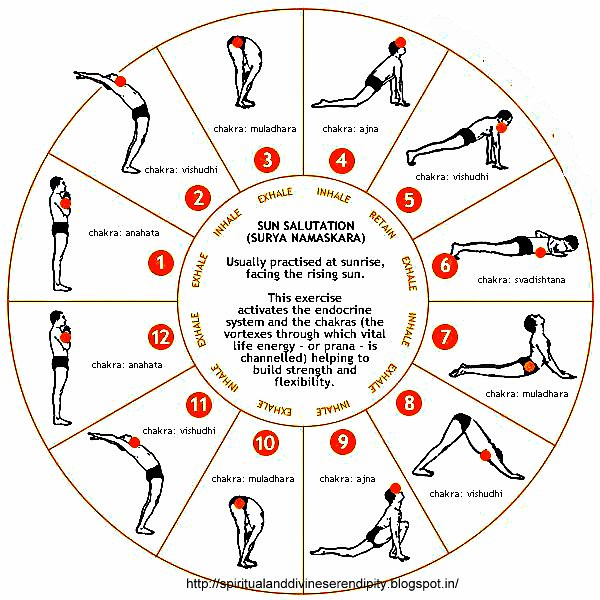The image is an artistic diagram resembling a circular wheel that outlines a sequence of 12 different yoga poses, each illustrated by a black and white figure. The diagram starts at approximately 10 o'clock with Pose Number 1, labeled "Chakra Anahata," accompanied by the instruction to exhale. The sequence continues clockwise, with each pose sequentially numbered and named after different chakras (e.g., Chakra Vishuddhi for Pose Number 2, Chakra Maladhira for Pose Number 3, and so forth). The final pose, Pose Number 12, returns to "Chakra Anahata" with the instruction to exhale again.

In the center of the wheel, the text reads: "Sun Salutation (Surya Namaskara)," usually practiced at sunrise facing the rising sun. This exercise is noted for activating the endocrine system and chakras—the energy vortexes through which vital life energy, or prana, flows—thereby helping to build strength and flexibility. The diagram also includes a URL at the bottom linking to "http://spiritualanddivineserendipity.blogspot.in".